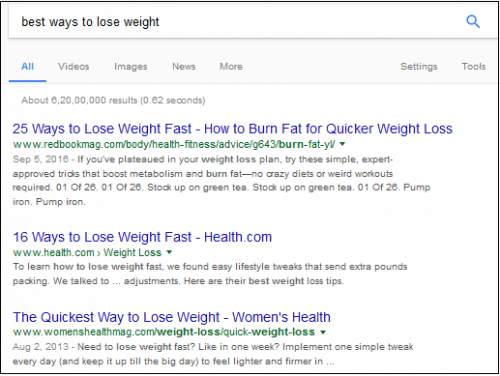This is a detailed screenshot of a Google search results page. At the top of the page, a white search bar prominently displays the phrase "Best Way to Lose Weight" entered into it. To the right of the search bar is a blue magnifying glass icon indicating the search function. 

Directly below the search bar, there's a navigation menu featuring various filter options. On the left side of this menu, there are five options: "All," "Videos," "Images," "News," and "More." On the right side, "Settings" and "Tools" are the available options. All the menu items are in gray, except for "All," which is highlighted in blue with an underline, indicating it is the selected filter.

Underneath the navigation menu, the search results section begins with text that states approximately "6,20,20,200 results," highlighting the vast number of related pages available.

Three main search results are visible:
1. **25 Ways to Lose Weight Fast** - This link caption remarks the topic of burning fat for quicker weight loss.
2. **16 Ways to Lose Weight Fast** - This result is attributed to Health.com.
3. **The Quickest Way to Lose Weight** - This link is associated with Women's Health.

The screenshot provides an organized and detailed view of the initial search results for methods to lose weight effectively.